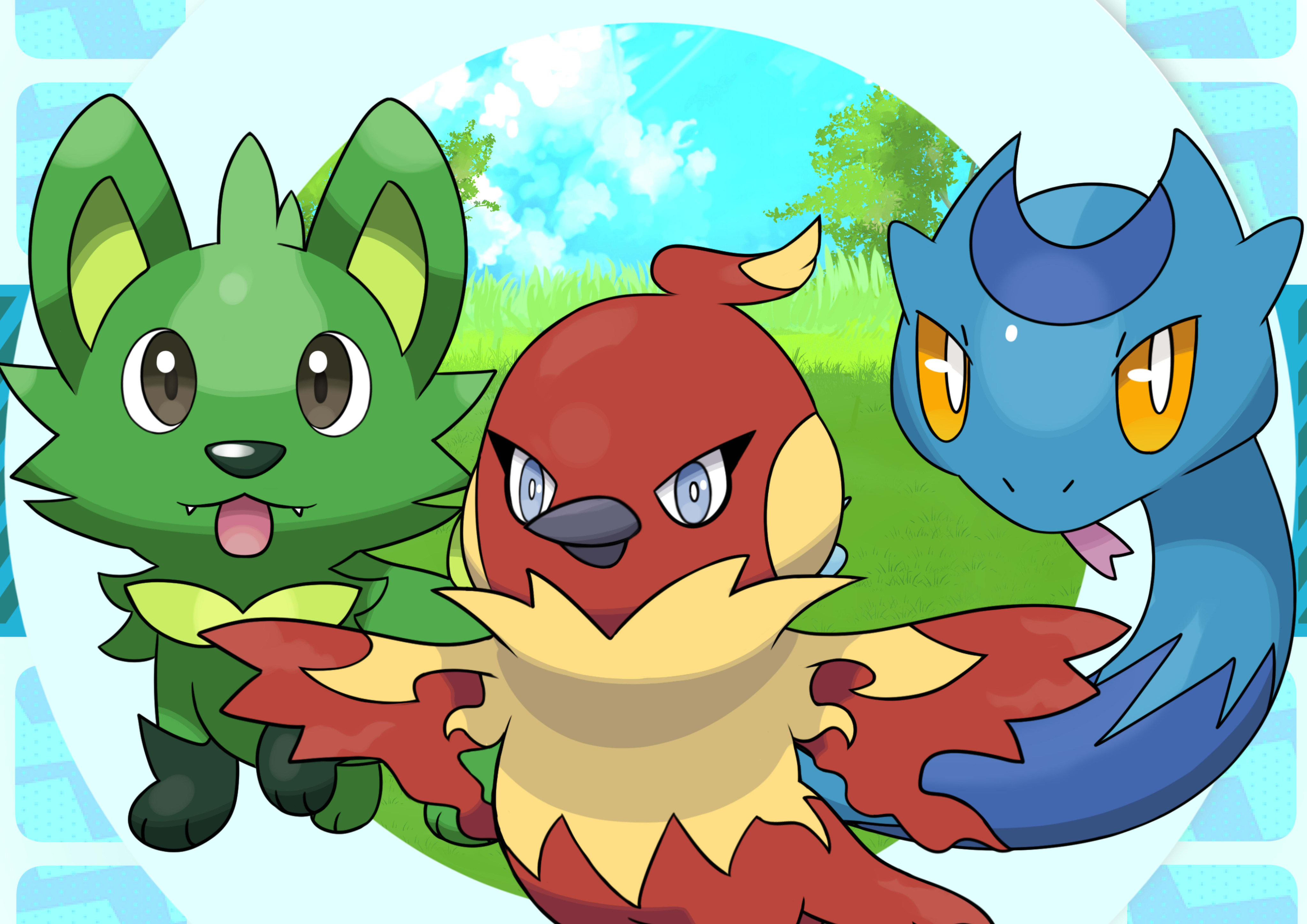This vibrant and meticulously detailed drawing showcases three captivating, Pokémon-inspired characters, imbued with a distinctly Japanese artistic influence. 

On the left stands a charming green dog with expressive, wide eyes and a playful red tongue peeking out. This creature sports black front paws and a pronounced black nose, while the inner part of its ears and a crest on its chest glow a bright yellow.

Central to the composition is a striking red bird, its wings elegantly outstretched. The bird's plumage features a harmonious blend of red and yellow hues, complemented by piercing blue eyes and a sharp black beak. A distinctive yellow tuft crowns its head, and its vibrant yellow chest flares majestically around its chin.

To the right slithers a serpentine blue snake adorned with a crescent moon marking on its head. Its piercing yellow eyes enhance its enigmatic appearance, with lighter blue scales on top blending into a darker blue underside.

The backdrop is a picturesque landscape framed within a circular white ring, revealing lush green grass and trees beneath a clear blue sky dotted with fluffy white clouds, adding a serene and natural ambiance to the scene.